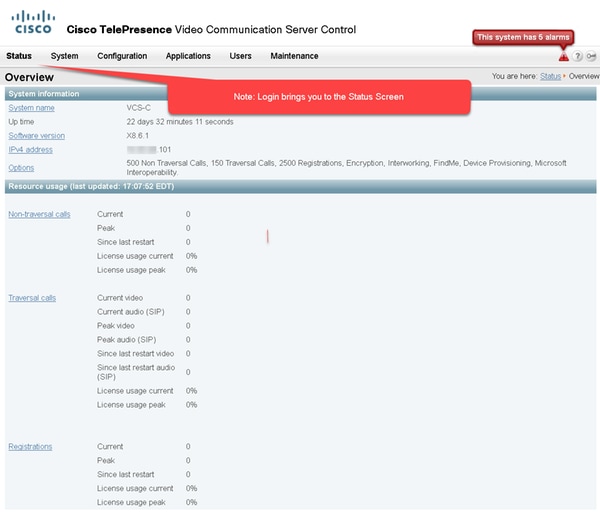The image depicts a user interface for Cisco TelePresence Video Communication Server Control. In the upper left corner, a series of small vertical lines are present, with the text "CISCO" in all capital letters positioned below them. Adjacent to this, the full title "Cisco TelePresence Video Communication Server Control" is displayed. Beneath this title, a long gray navigation bar extends horizontally, offering several menu options: Status, System, Configuration, Applications, Users, and Maintenance.

On the left side of the interface, under the "Status" tab, there is a prominent red box containing a long red line. Inside this box, a note is displayed, informing the user that "Login begin brings you to the status screen."

In the upper right corner of the interface, another red box stands out, which notifies the user that "The system has five alarms," accompanied by a black exclamation point inside a red triangle symbol.

Further down the interface, a blue box highlights "Resource Usage" with the latest update timestamped as "Last updated 1707-52 EDT." Below this section, three categories are listed vertically and underlined: Non-Transit Calls, Traversal Calls, and at the bottom, Registrations, also underlined and in blue.